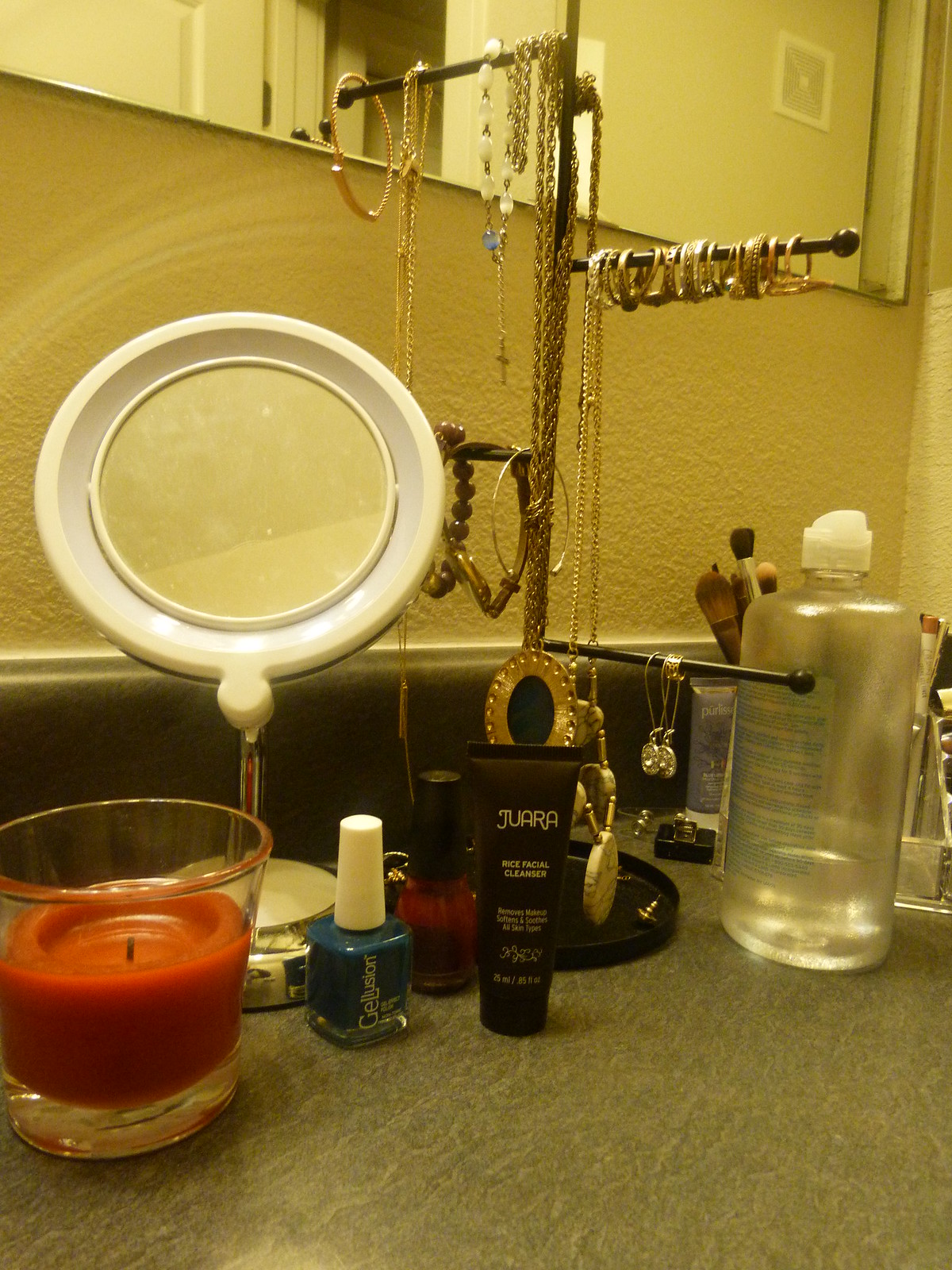The image depicts a bathroom counter adorned with a variety of personal items. At the center stands a "jewelry tree," gracefully organizing several pieces of jewelry. One arm holds a collection of rings, while two other arms are draped with an assortment of bracelets. Longer pieces, including necklaces, hang elegantly from the remaining branches, with a notable cross on a chain catching the eye. Scattered around the base of the jewelry tree are various makeup products, including bottles of nail polish and what appears to be a jewelry cleaner. A mirror with a circular, fluorescent light framing its edges is positioned nearby, enhancing visibility. In the background, a cluster of makeup brushes stands ready for use. An orange-colored candle encased in glass adds a warm, inviting touch to the scene. Additionally, a bottle containing a clear liquid is present, adding to the assortment of personal care items.